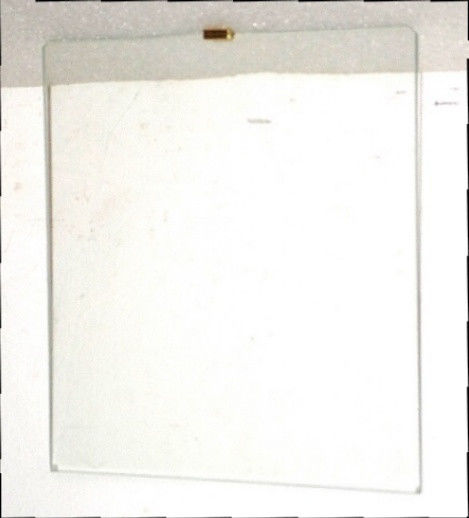The image depicts a slightly rectangular whiteboard with a bulky, somewhat grown-out frame that gives it a sunken appearance. Dominated by various shades of white, the whiteboard has a used look, with multiple marks scattered across its surface. Centered at the top of the board is a small black object, likely a brush used for erasing writings, adding a touch of detail against the predominantly white and light gray background. A bronze or dark brown hue is observed around the edges, possibly hinting at the frame or surrounding elements. The minimalist and color-muted scene suggests the whiteboard is resting on a flat surface, perhaps a table.